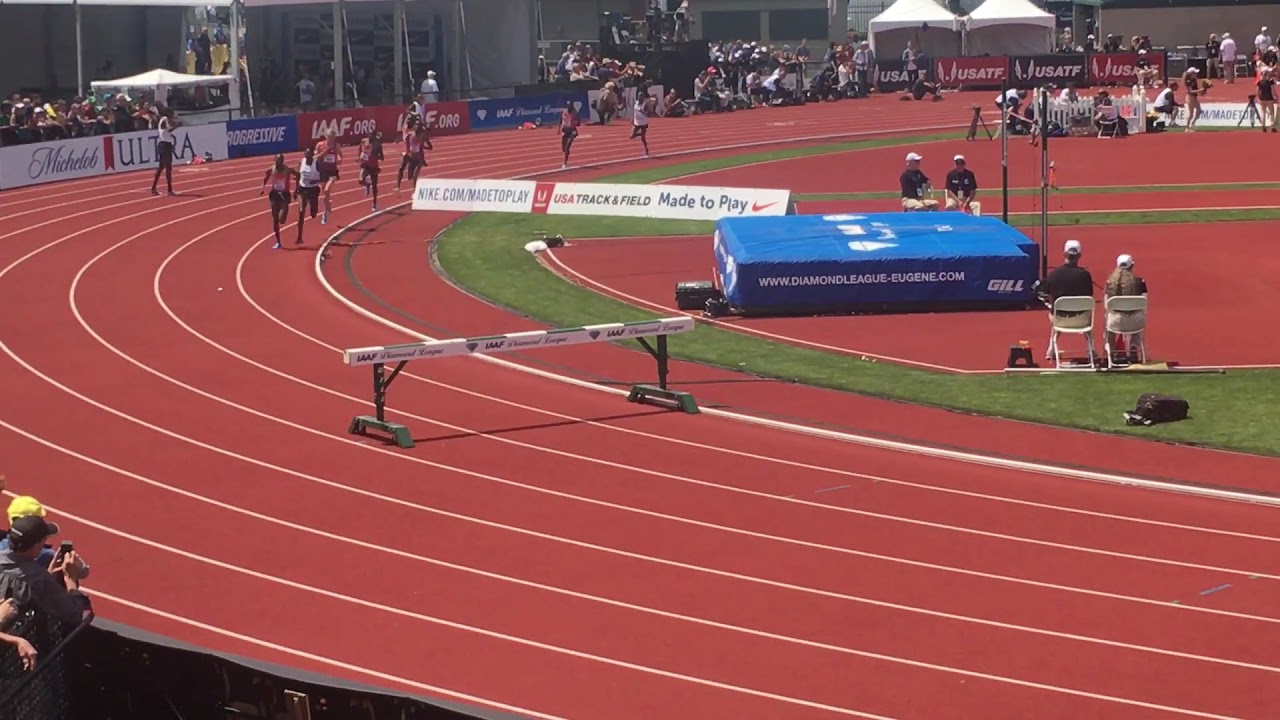The photograph captures an outdoor track and field event, likely hosted by the USATF (United States of America Track and Field Organization), as signified by multiple signs with the USATF logo in black and red. The track surface is a vivid red, marked with white lane stripes, and runners in red and white jerseys are visible, rounding a corner on the left side of the track. A hurdle is set up on the track, indicating a race involving obstacles. Surrounding the track are green grass areas, sections for the high jump in red, and some white fencing. Spectators line the edge of the track, many equipped with cameras, with more attendees seated in the stands across the field, including notable figures like a person in a black baseball hat and another in a yellow hat. Advertisements are prominently displayed, including banners for Michelob Ultra, Progressive, IAAF.org, and several others. Central to the scene are signs stating "nike.com/made to play" alongside "USA Track and Field," with the recognizable red Nike swoosh logo. White tents are also visible in the background, adding to the bustling atmosphere of the event.